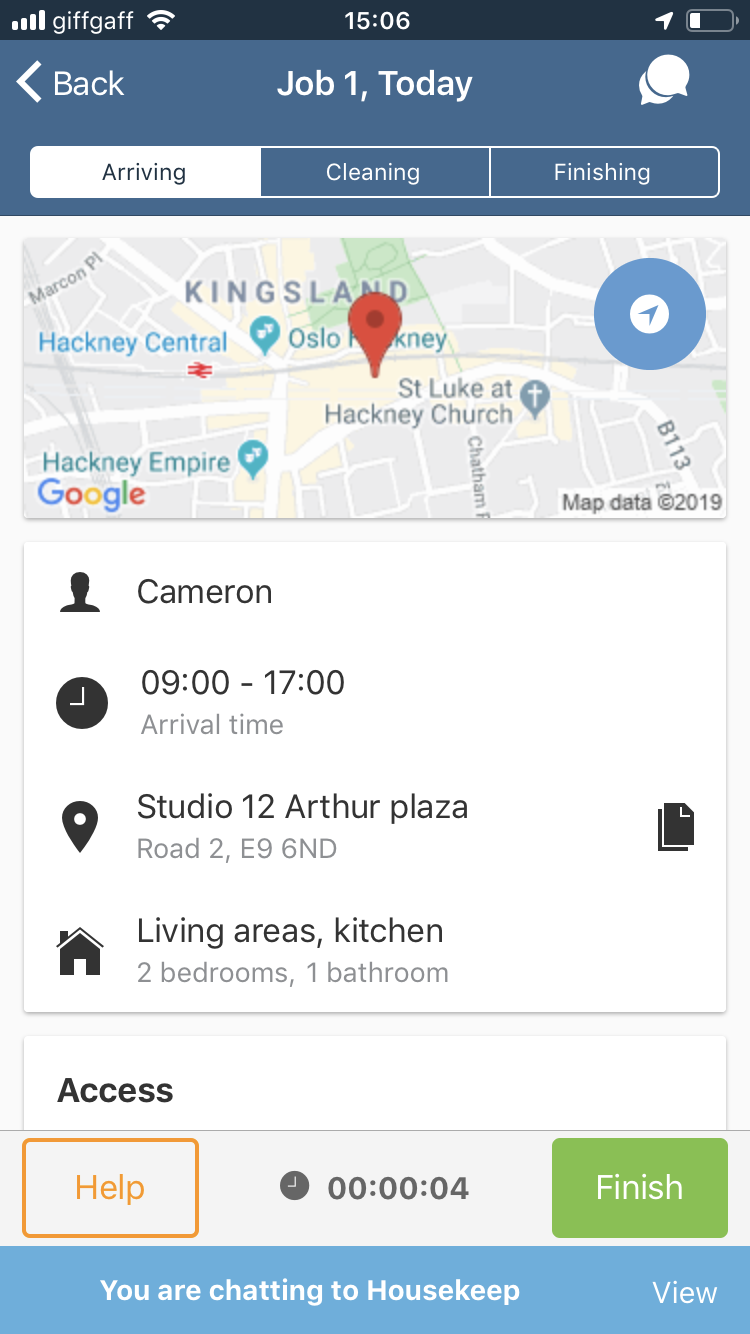**Detailed Descriptive Caption:**

This image is a screenshot of a map or navigation application, primarily showing a map in the upper portion. Centrally placed on the map is a prominent red button. To the right of the red button, there is a prominent circular icon with a blue background. Nested within this blue circle is a smaller, white circular icon featuring a blue arrow pointing toward the upper right corner of the image.

In the top right corner, there is a battery icon in dark gray, indicating a low power level of approximately 10 to 15 percent, signified by a narrow white bar. Adjacent to the battery icon, the current time is displayed as "15:06" in white text, set against a dark blue horizontal header background.

Beneath the map, there is detailed information regarding the current destination. This includes several icons and corresponding text on the left side. The first icon is a silhouette of a person's head and shoulders labeled "Camera." Below this, a circular clock icon with white hands indicates an arrival time between 09:00 and 17:00 hours. Further down, an address is provided, though the specific text is not fully visible here. The final icon on this list is a black house, representing details about the destination property, which is noted to have "2 bedrooms and 1 bathroom" in light gray text.